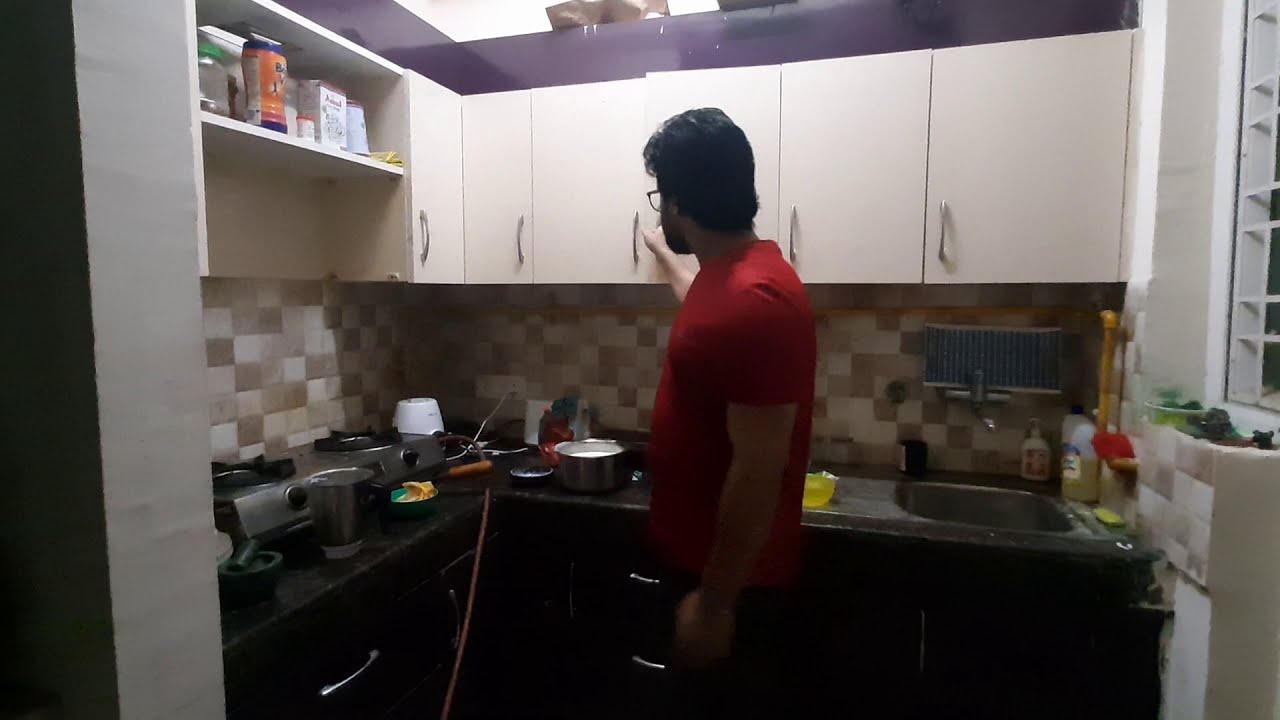In the image, there is a man with short, neatly maintained black hair, a beard, and wearing dark-framed glasses and a red t-shirt paired with black trousers. He is standing in a well-appointed, L-shaped residential kitchen that features a blend of white, tan, and brown tiles on the backsplash. The kitchen has white cabinets above dark, marble-like countertops and black lower cabinets with silver handles. The man is turned slightly away from us, reaching with his right hand towards an upper cabinet handle, while his left hand rests by his side. The countertop surface holds various items, including a portable gas stove, a cup, a saucepan, and a yellow bowl. To the far right is a small sink area accompanied by dish soap. A window is located on the right side of the image, adding light to the compact and organized kitchen space.